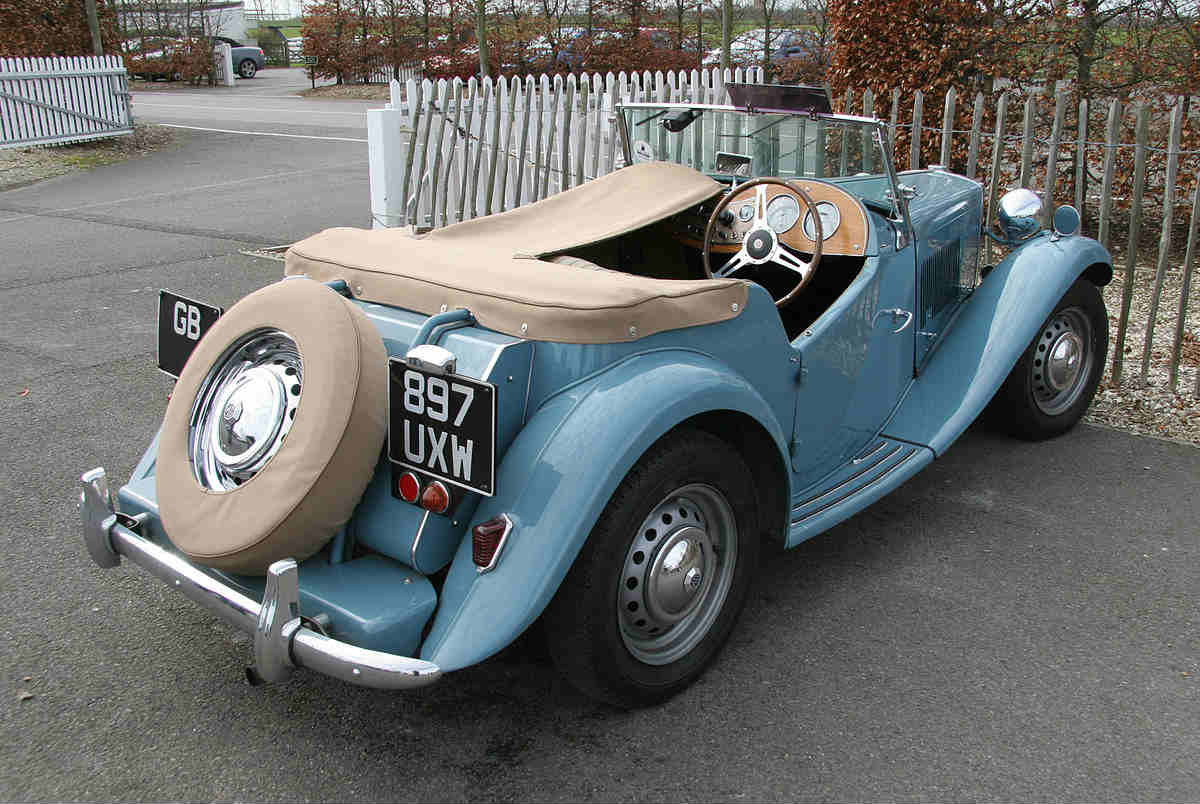This is a daytime color photograph prominently featuring a vintage convertible automobile from the 1940s or 1950s, positioned centrally in a small parking lot. The classic vehicle, likely a roadster, is distinguished by its curvy design and eye-catching baby blue body with a tan leather cover concealing the convertible area and a similarly covered spare tire mounted on the back, flanked by shiny silver hubcaps and a bumper. The license plate reads "GB 9897 UXW". The car, with its driver's seat on the right side, faces inward against a small wooden fence. Above this fence, the background reveals green trees and some more modern cars. Colors in the image span lighter bluish gray, tannish gray, black, white, red, darker red, reddish-orange, and a bright greenish-gray, creating a vivid and nostalgic scene.